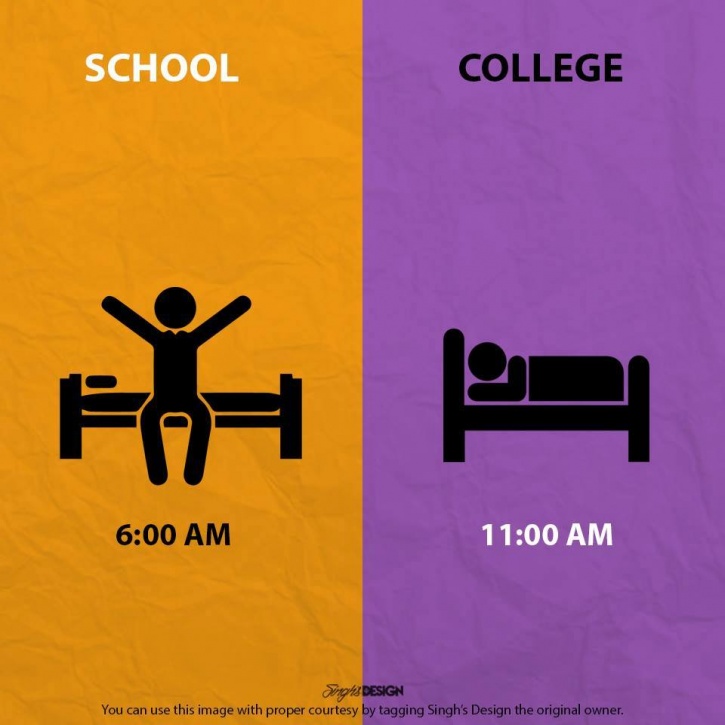The image is a humorous comparison of wake-up times for "school" and "college," divided into two sections. The left half, with an orange background, is labeled "SCHOOL" in white, uppercase letters at the top. Beneath it, there's a simplistic icon of a person sitting up in bed with arms stretched out, and below them, "6 a.m." is written in black. The right half features a purple background and is labeled "COLLEGE" in black text at the top. This section shows the same person lying in bed, still asleep, with "11 a.m." written in white text beneath the bed. The overall design highlights the stark contrast in wake-up times, suggesting early mornings for school and late mornings for college. The image credits at the bottom mention "signs, design," indicating proper courtesy for usage.